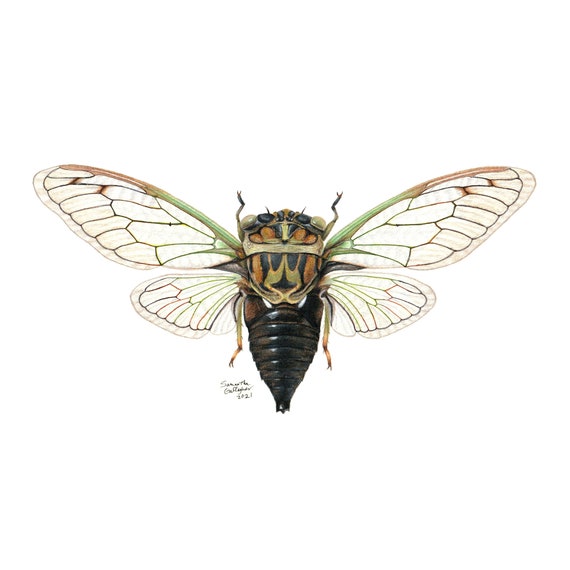A vivid and intricate illustration of an insect can be seen in this image, resembling either a fly, bee, or dragonfly in appearance. The insect is positioned with its head pointing upwards and appears to be almost lying on its back. Its head is shield-shaped and multicolored, featuring shades of reddish-brown, dark gray, and lighter green, with conspicuous face-like features including optical illusions of eyes and an open mouth. The head tips with additional exaggerated compound eyes, arranged with two inner black circles and two outer white circles.

The body of the insect tapers and is segmented with horizontal ridges, colored in a reflective black that creates a polished effect. Extending from the head section are two large, transparent wings on each side with intricate geometric patterns framed in black and green hues. These wings show a stained-glass-like grid pattern and subtle color transitions from green to pink towards the edges. Behind the primary wings are two smaller wings exhibiting similar but less pronounced designs.

The insect's legs are arranged with two extending forward over the head and two more folded rearward, near the segmented hind part, which comes to a sharp point. The entire illustration is set against a stark white background, emphasizing the detailed artistry of the insect. Additionally, there is a barely discernible signature beneath the lower left leg with the year "2021" inscribed.